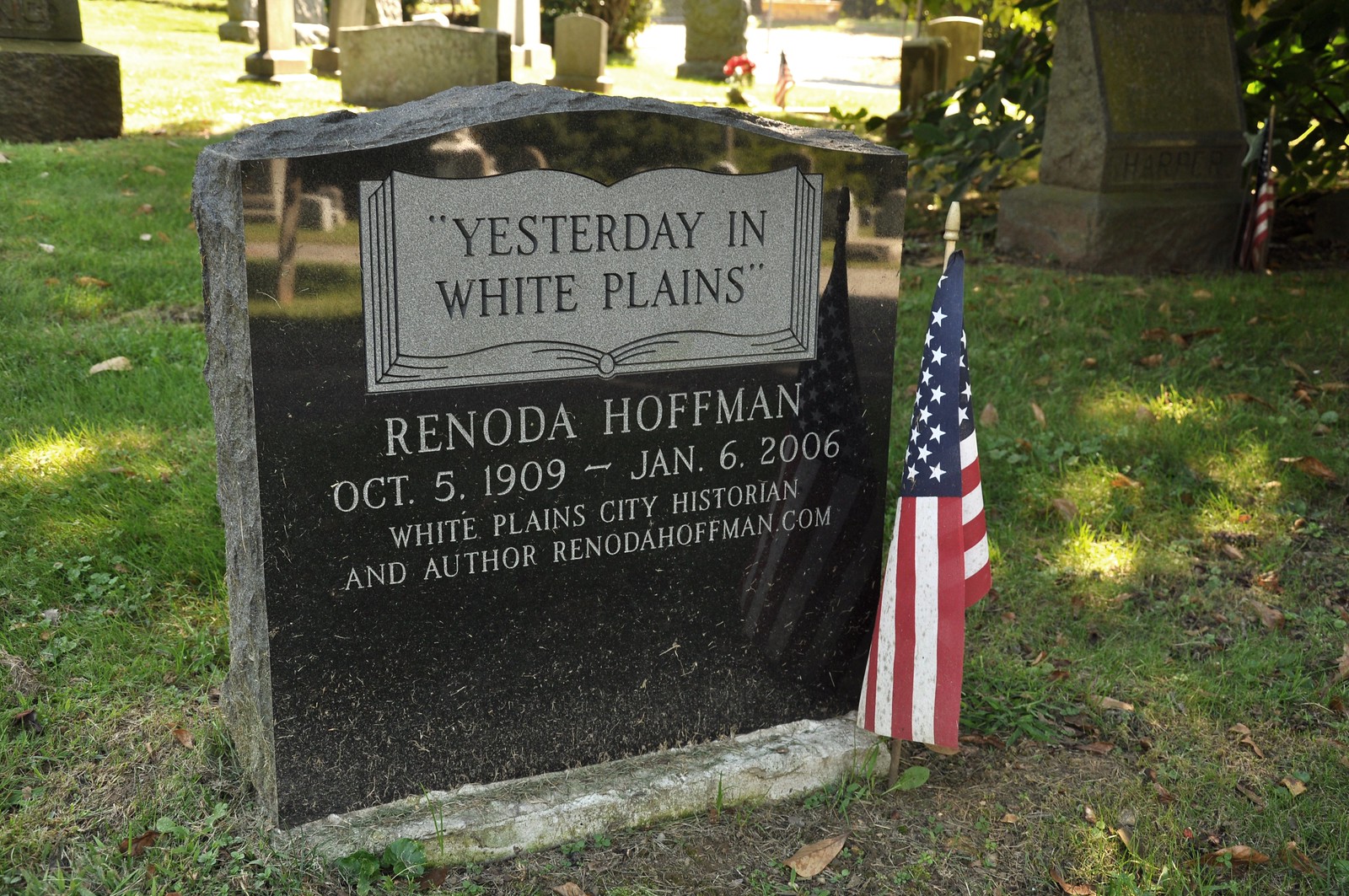In this full-color, horizontally rectangular photograph taken outdoors on a sunny day, we see a serene cemetery scene. A smooth, black granite headstone dominates the foreground, with its surface polished to a reflective shine. The top of the stone features a distinctive small curve with natural rock indentations, creating a beautiful contrast with the smooth lower portion.

Etched in light gray on the headstone is what appears to be an open book design bearing the quote, "Yesterday in White Plains." Below the quote, the details read: Renota Hoffman, October 5, 1909 – January 6, 2006, White Plains city historian and author, along with her website, renotahoffman.com. 

A small American flag is placed respectfully next to the headstone. In the background, under the bright midday sun, you can see a well-maintained grassy area scattered with tombstones, vibrant red flowers, and another American flag fluttering in the light breeze, contributing to a peaceful ambiance. The sunlight streams down, casting a warm glow over the entire scene.